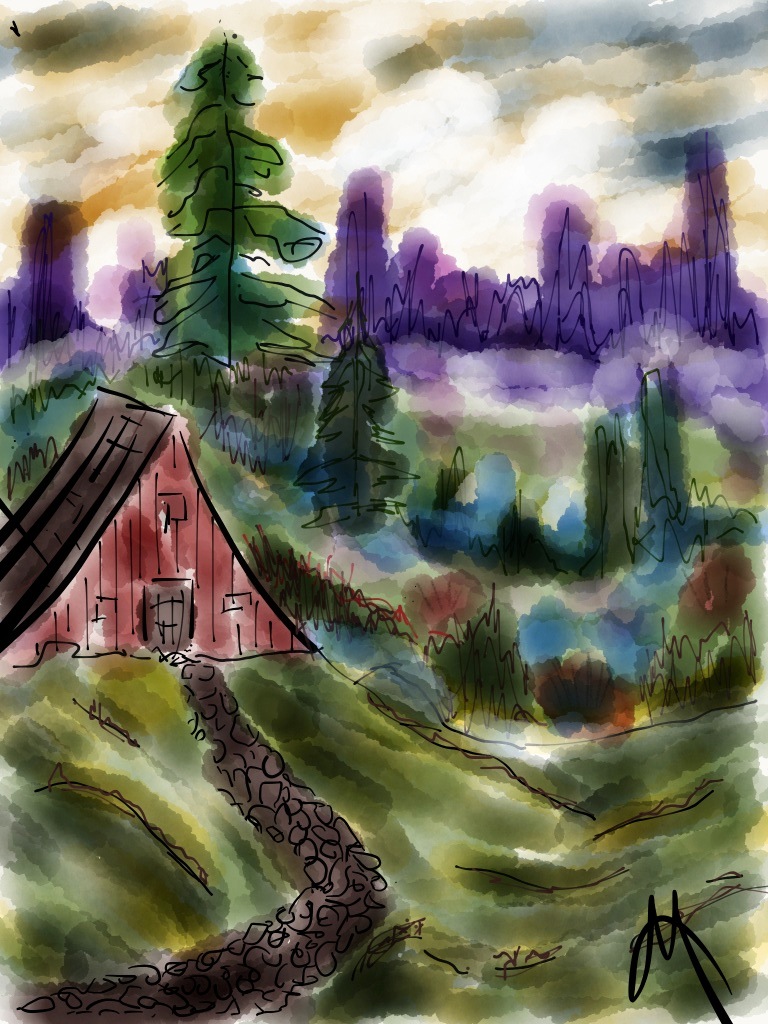This vertically oriented painting, rendered in gouache or watercolor with black pen and ink accents, depicts an A-frame building positioned slightly left of center. A winding path leads up to this structure, inviting the viewer into a captivating landscape scene. In the foreground, rolling hills undulate into the background, creating depth through a series of overlapping sections. Vertical trees punctuate the composition, including a distinctive line of purple trees that recedes into the distance. The sky above is blotchy, with swirling paint strokes that add dynamic texture to the scene. The artist employs a rich color palette of reds, greens, browns, blues, purples, and yellows, blending harmoniously to evoke a vivid and lively atmosphere. The painting is signed in the bottom right-hand corner with an elegant, cursive capital letter 'M'.